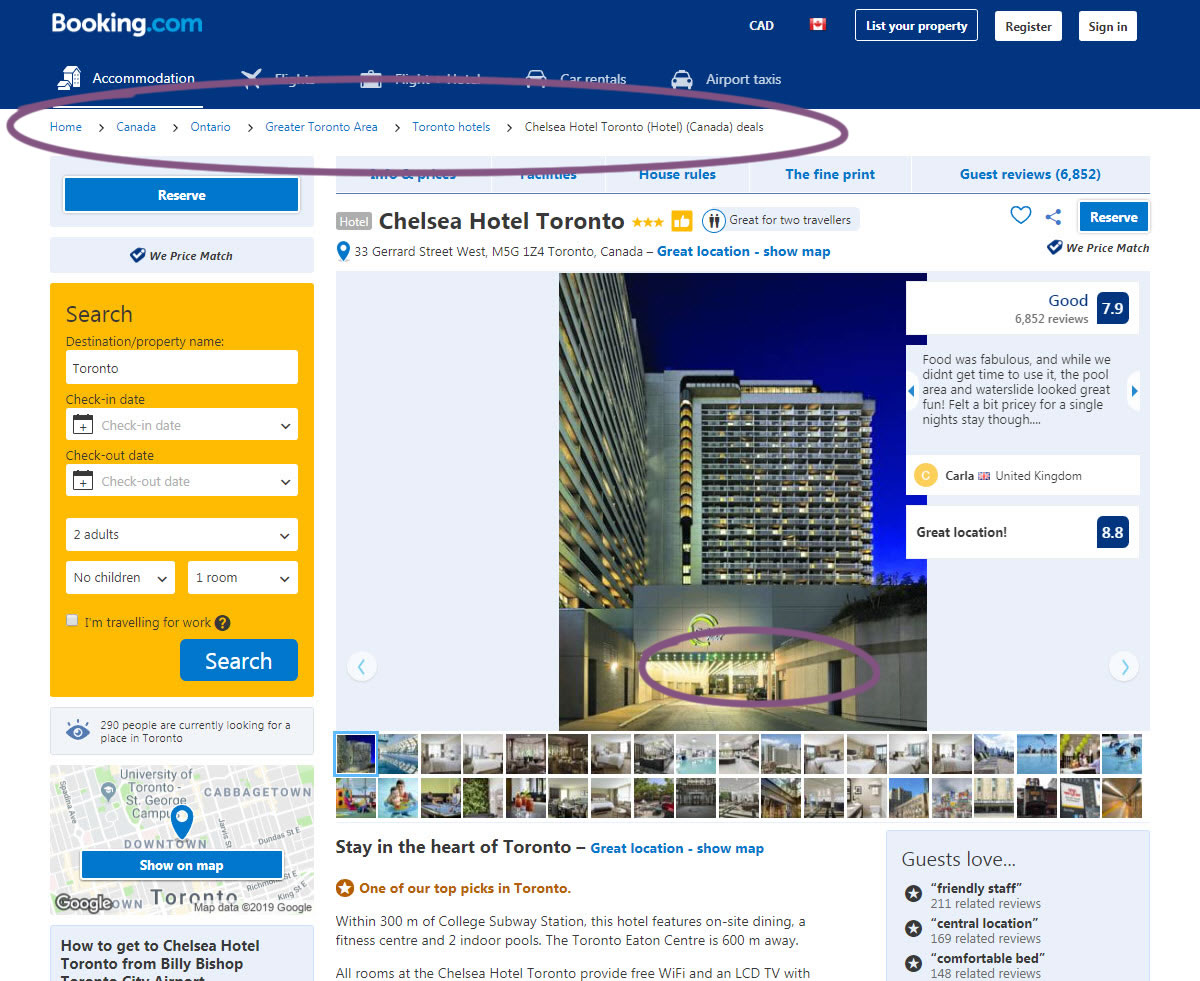The image appears to be a screen capture from a tutorial on how to book a hotel using the website Booking.com. The tutorial seems to specifically reference the Chelsea Hotel in Toronto. Elements highlighted in the tutorial include a series of steps encircled to guide the viewer through the booking process. The Chelsea Hotel is a large and tall structure with at least 20 floors. The main image is of the hotel, which shows what appears to be the entrance or a side entrance circled for emphasis. Surrounding this primary image are numerous smaller thumbnail images, presumably showcasing different aspects of the hotel, which can be clicked to view in the main display area. In the upper left of the screen, there is a search bar where "Toronto" has been entered, and the selection indicates a search for accommodations for two adults. The overall layout of the screen capture suggests a detailed walkthrough aiming to assist users in selecting and booking a hotel room on Booking.com.